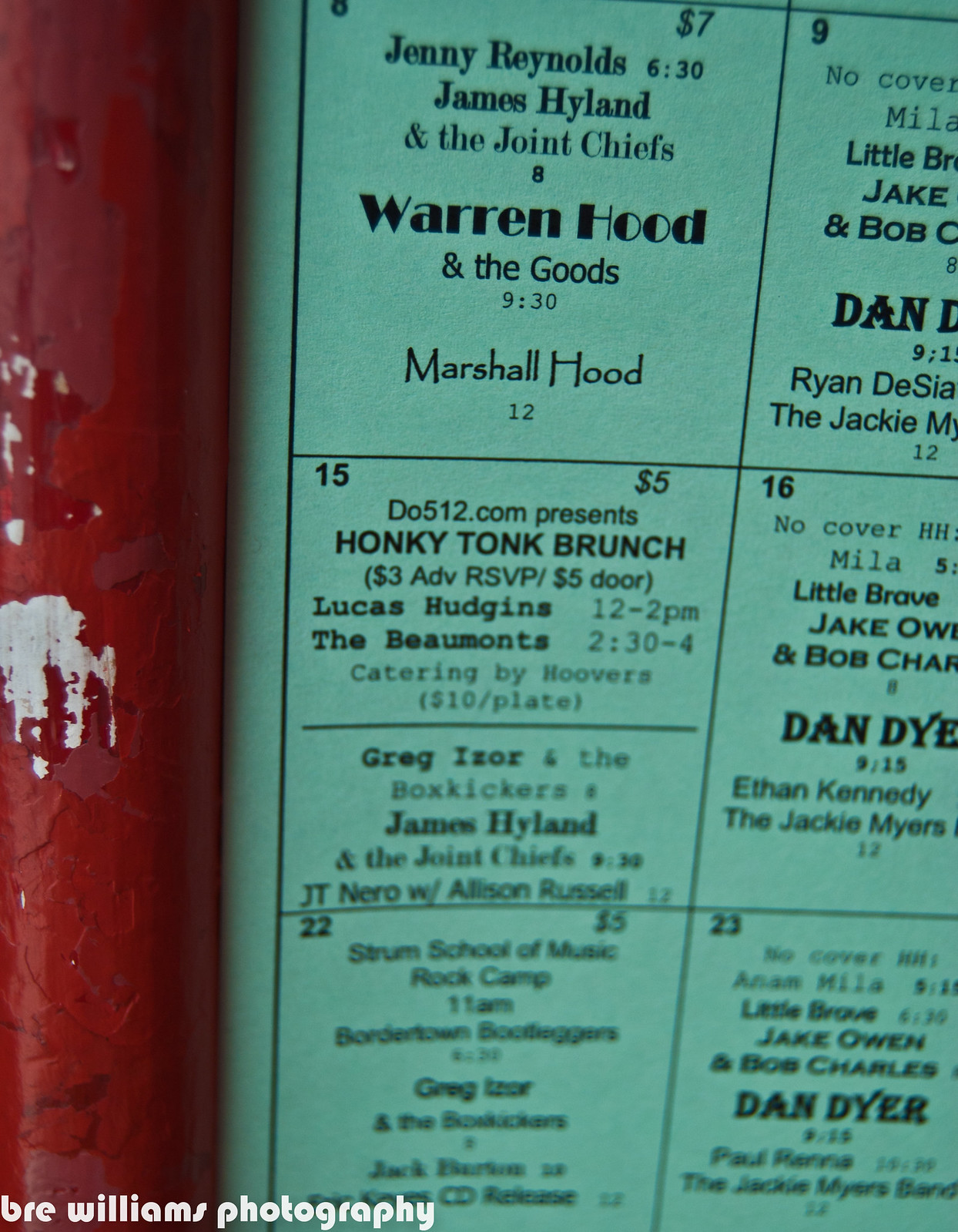The image depicts a part of a calendar set against a Tiffany blue or green background interspersed with various squares, resembling a checkerboard pattern. Each square contains event details with numbers indicating dates in the top corners, performer names centered, and times and dollar amounts noted at specific positions. Among the visible dates, for the 8th, it lists performances by Jenny Reynolds at 6:30 PM, James Highland and the Joint Chiefs, Warren Hood and the Goods at 9:30 PM, and Marshall Hood. The 15th includes a Honky Tonk Brunch, and the 16th features events like Little Brave, Jake Owens, and Bob (cut off). On the 22nd, there is Strum School of Music Rock Camp, and on the 23rd, mostly cut off or blurry, the name Dan Dyer is visible. Text such as "Bree Williams Photography" is displayed in white at the bottom left. To the left of the calendar, there is an indistinct red object, possibly wood or metal, with some chipping exposing a white layer underneath. Additionally, mentioned details include Lucas Hudgens performing from 12 to 2 PM and the Beaumonts from 12:30 to 4 PM, with catering by Hoover's at $10 per plate. The calendar serves as a detailed schedule of musical performances and events, with some elements being partially obscured or cut off.